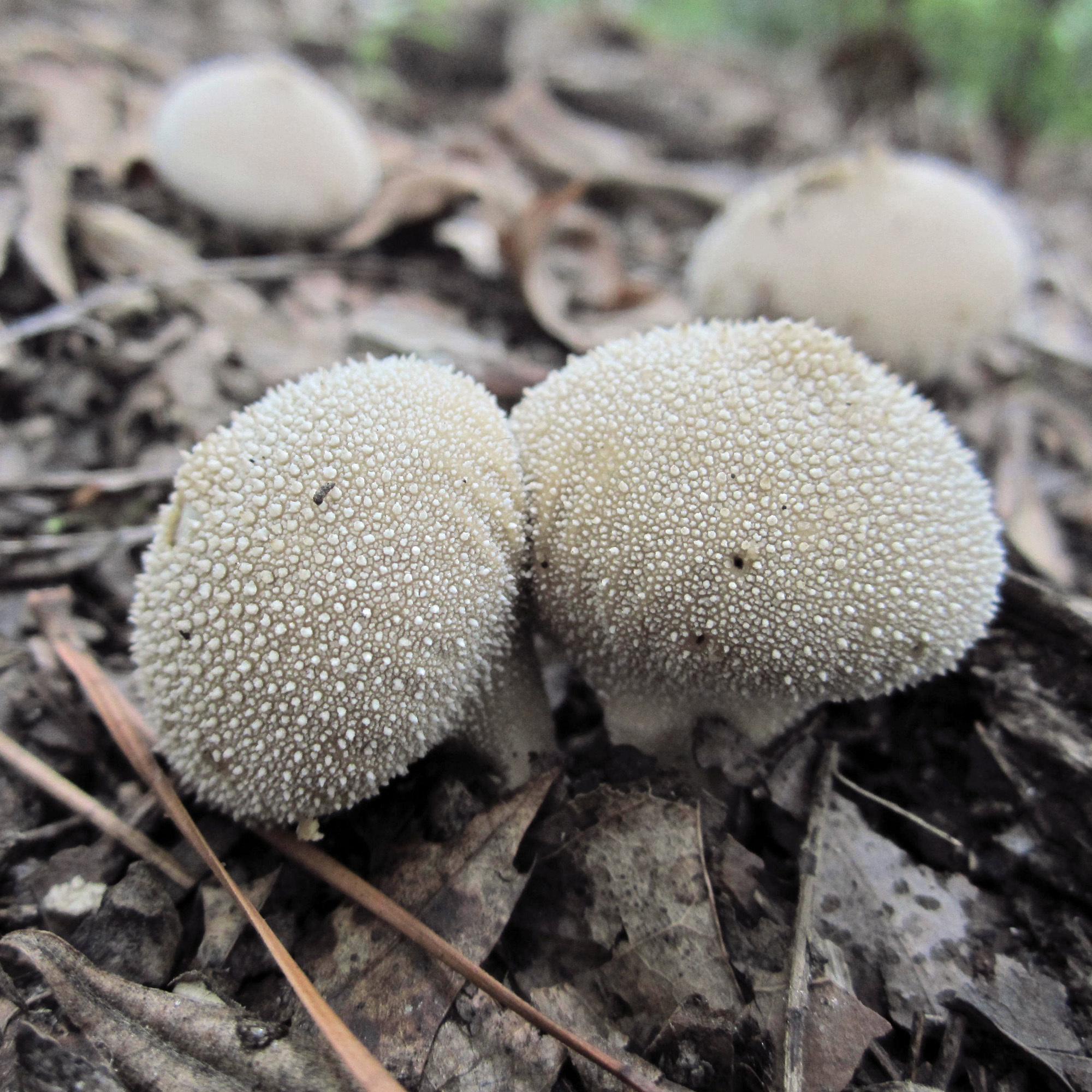The image depicts a nature scene showing four unusual, tan-colored mushrooms emerging from a bed of dead leaves and dirt. In the foreground, two of these mushrooms are shown in close-up detail, displaying a unique bumpy texture with soft, flexible-looking points. They appear to be pushing against each other, almost as if one is nudging the other aside. In the background, two more mushrooms can be seen, although they are blurred and appear to have smoother caps compared to those in the foreground. The setting appears to be a forest floor, given the abundance of natural debris and a patch of green grass visible beyond the immediate area. The image has been modified to enhance contrast and shadows while reducing saturation, giving the mushrooms an almost dangerous, potentially poisonous appearance. This detailed photograph highlights the eerie yet fascinating nature of these fungi, making it a striking composition of the forest undergrowth.